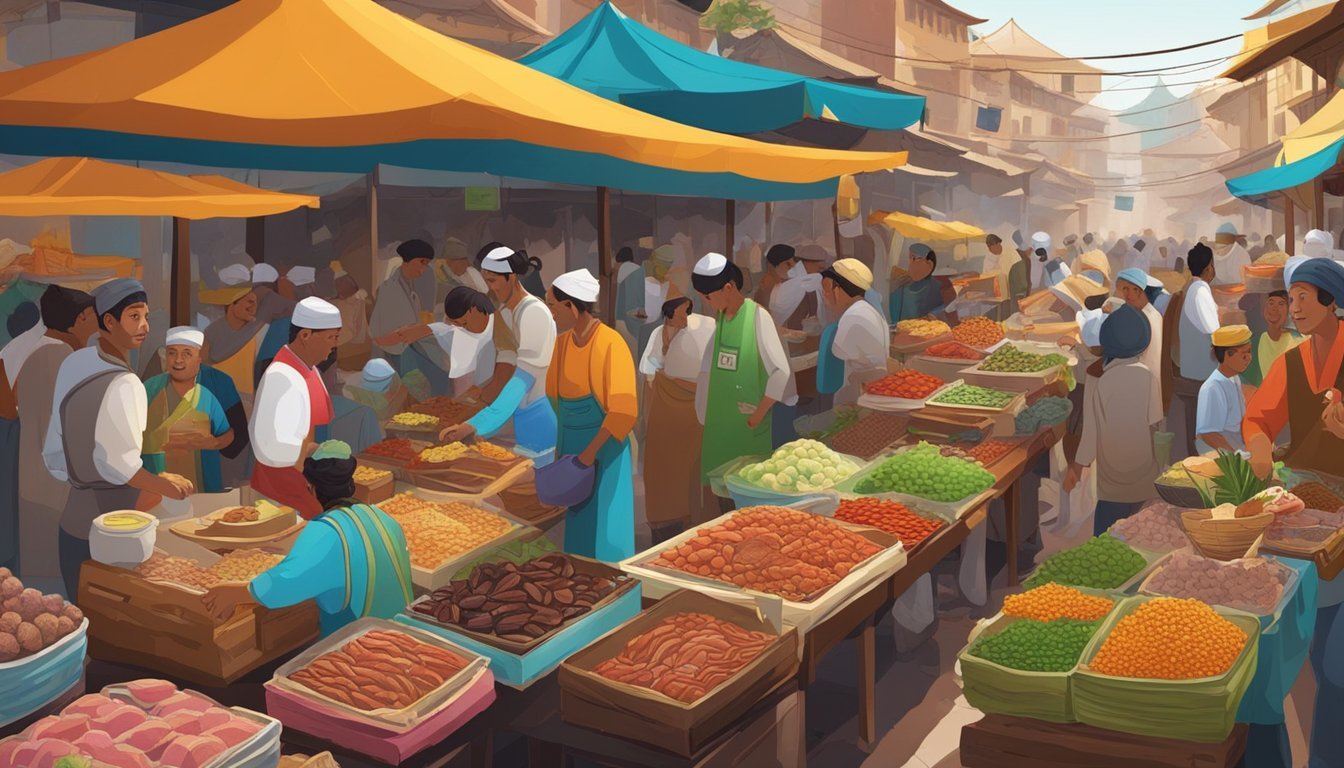The image depicts a vividly stylized painting of an open-air market, likely set in the Middle East, as suggested by the distinct architecture and the white clothing worn by the numerous brown-skinned people. The market scene is bustling, with vendors selling a variety of foods, including green and orange beans, red beans, Brussels sprouts, coffee beans, and meats. The crowd wears a mix of white tunics, shirts, and hats, which are typical in desert climates to combat the sun, as well as colorful aprons and garments in hues of orange, red, and green, adding vibrancy to the scene. The market is set against a backdrop of buildings with several floors and yellow and blue tents covering the street. Lines are strewn between the buildings, enhancing the lively, immersive atmosphere, with countless figures receding into the background, indicating the market's extensive scale.